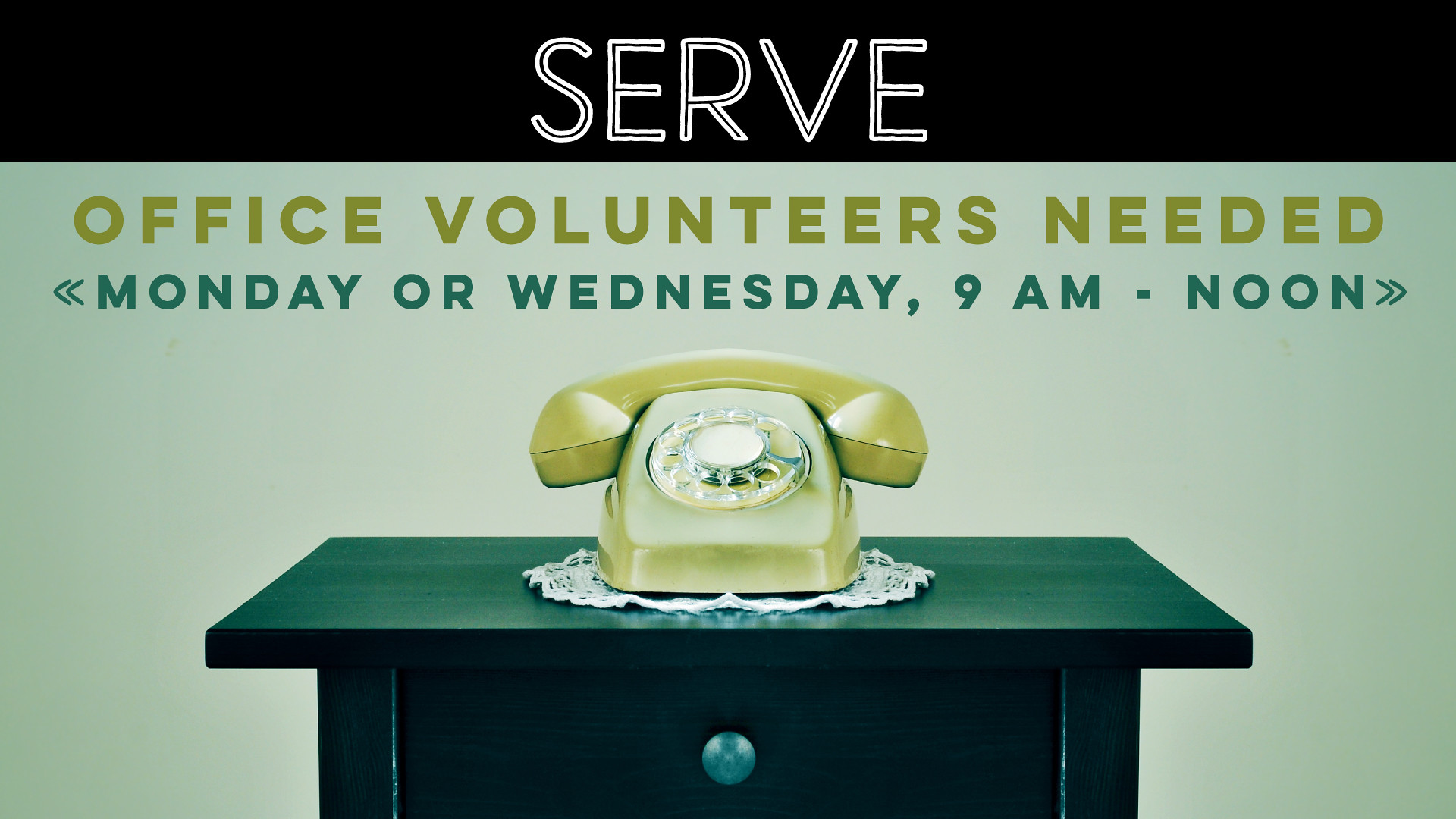The image is a detailed advertisement calling for office volunteers. At the very top of the advertisement, there is a black banner with bold white capital letters that read "SERVE." Below that, in a dark green font, the text states "Office volunteers needed," followed by "Monday or Wednesday, 9 a.m. - Noon" in green. The central focus of the image is a vintage yellow rotary telephone, resting on a white paper doily. The phone sits on a small, dark green piece of furniture, possibly a nightstand or an end table, which has a silver handle or knob in the middle of a small drawer. The entire setting is bathed in soft lighting with a slight greenish tint, enhancing the nostalgic feel of the scene.